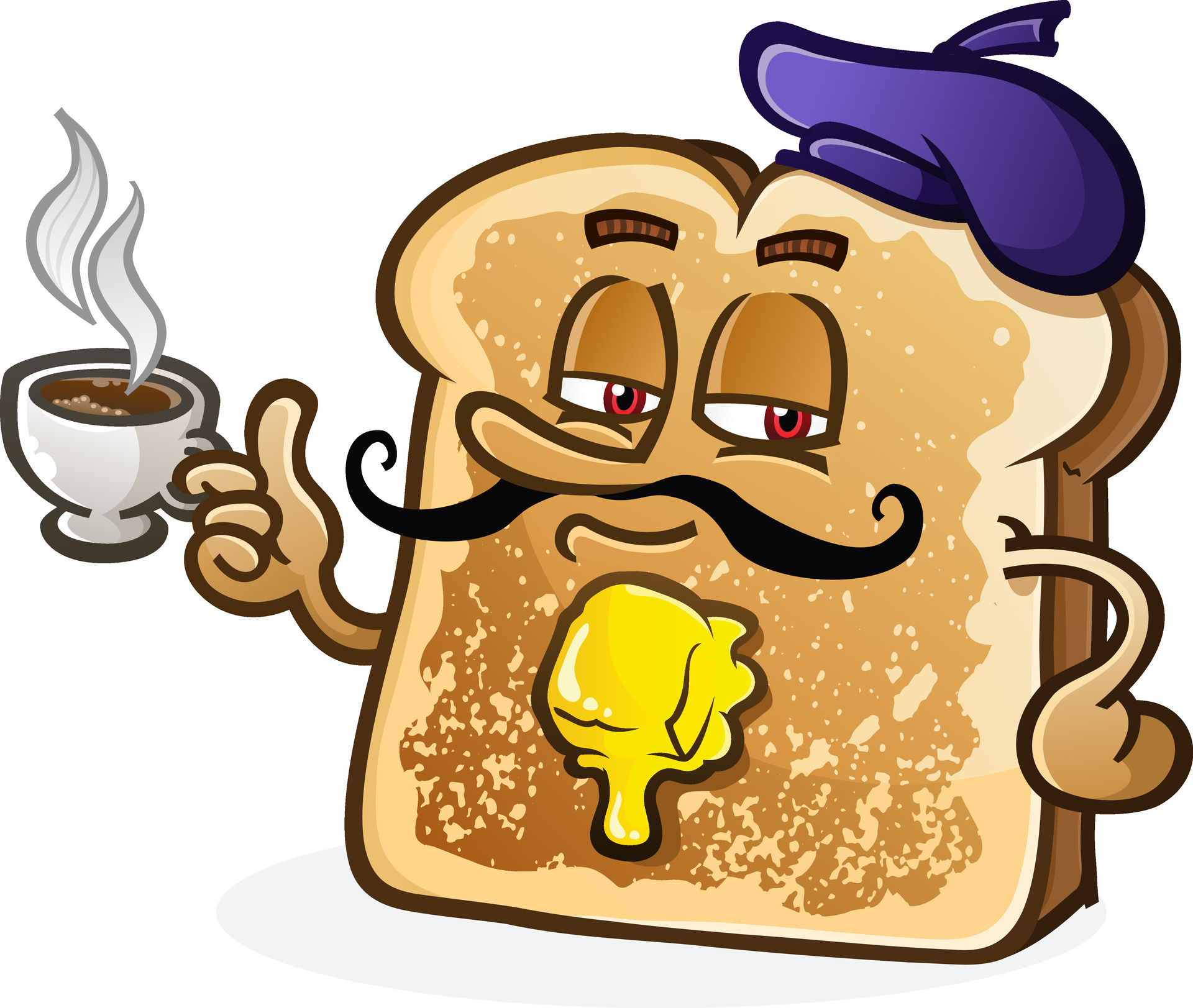The image depicts a comical and cute cartoon slice of toast. The toast, light brown with slightly darker edges, appears 'French' with a large Pinocchio-like nose, black curly mustache, and a purple beret perched on one corner of its head. Its eyes are striking with red pupils. Just below the mustache, there's a cartoon depiction of a pat of butter resembling a beard. This anthropomorphic toast has thin, brown arms ending in circular hands, with the right hand holding a white mug containing brown coffee, from which light gray steam rises. The background of the image is white, highlighting the quirky features of this toast character.